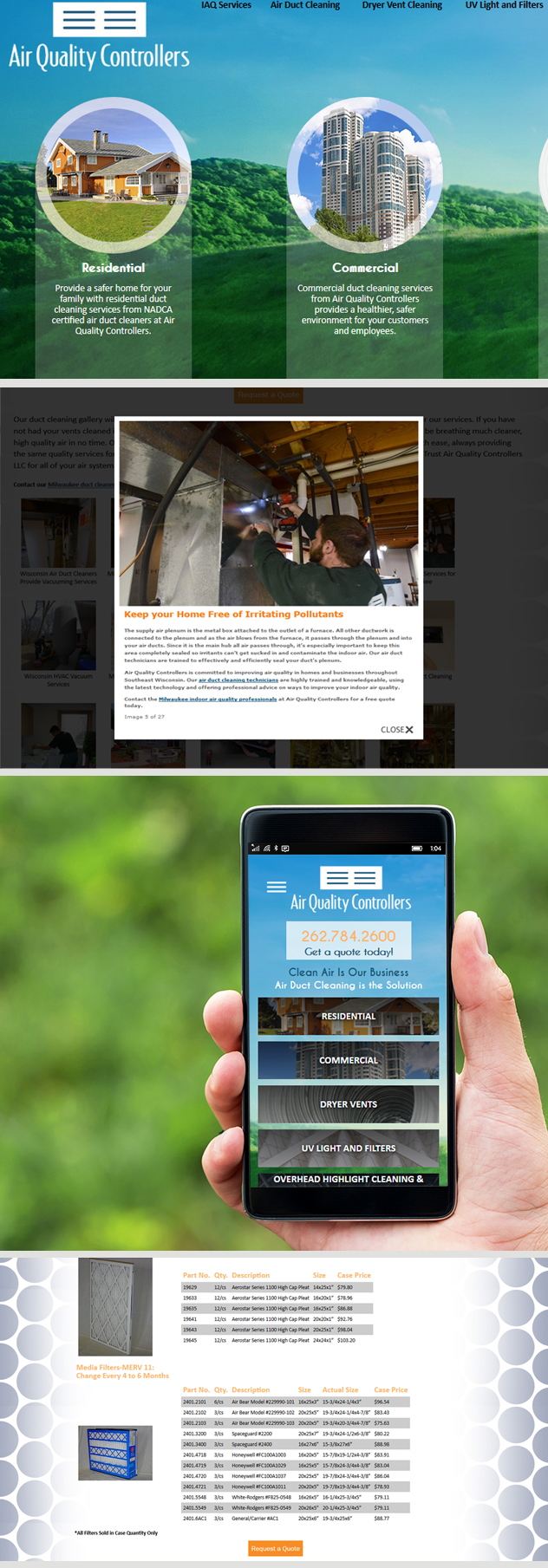The image at the top features a gradient background, starting with a bluish sky dotted with white clouds, transitioning into green hills, and then fading into a white section. At the very top, the text "Air Quality Controllers" is prominently displayed in black. Below this, the services offered are listed: "IAQ Services, Air Duct Cleaning, Dryer Vent Cleaning, UV Light, and Filters."

The image includes two distinct circles. The left circle features an Amish-style house with the caption "Residential: Provide a safer home for your family with residential duct cleaning services from NADCA-certified air duct cleaners at Air Quality Controllers." The right circle shows a modern white commercial building with green glass mirrors, captioned "Commercial: Commercial duct cleaning services from Air Quality Controllers provide a healthier, safer environment for your customers."

A white line runs across the image, above a pop-up featuring a man using a red and black drill, accompanied by the tagline "Keep your home free of irritating pollutants."

Further down, the text becomes blurry, revealing two paragraphs in black with some sections underlined in blue. Below this, there's a somewhat blurry picture with a green background, showing a person holding a black phone. The website information is displayed, including the phone number "262-784-2600". In blue text, it states "Get a Quote Today" and "Clean Air Is Our Business". Additionally, there's a white section listing "Air Duct Cleaning Solutions, Residential, Commercial, Dryer Vents, UV Light, Overhead Cleaning, Highlight Cleaning."